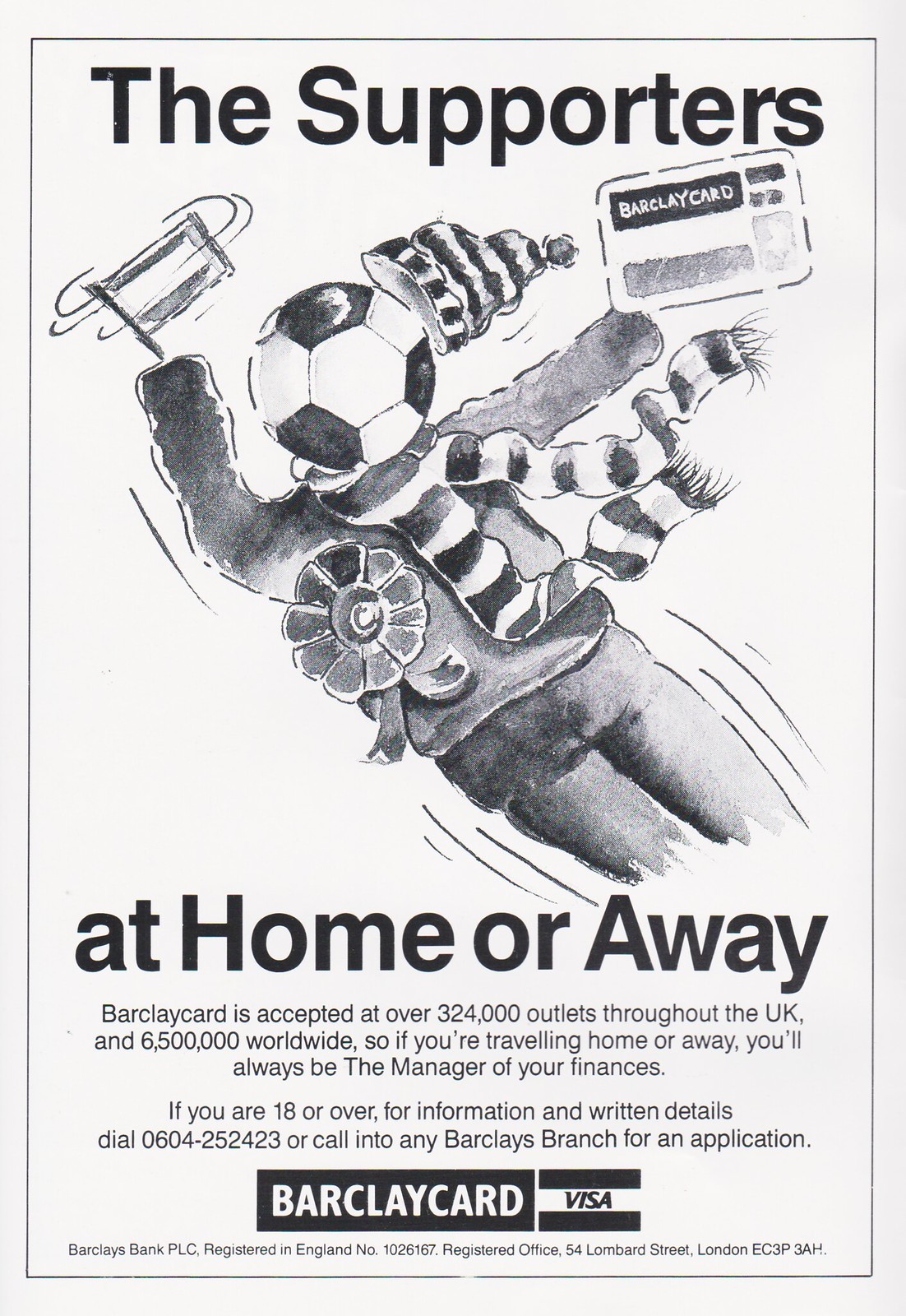This vintage-styled black-and-white ad from a football club program features an eye-catching illustration of a fan with a soccer ball for a head. Titled "The Supporters," it showcases the fan in motion, waving a flag and adorned with a striped scarf and a snow hat. The fan also prominently holds a Barclaycard, highlighted by the surrounding text, "At Home or Away," emphasizing the card's wide acceptance. Listed below are the benefits of the Barclaycard, stating it is accepted at over 3,240 outlets throughout the UK and 6,500 worldwide, ensuring users can manage their finances effortlessly while traveling. The ad's design combines classic print publication elements with dynamic black-and-white illustrations to capture the essence of football fandom.